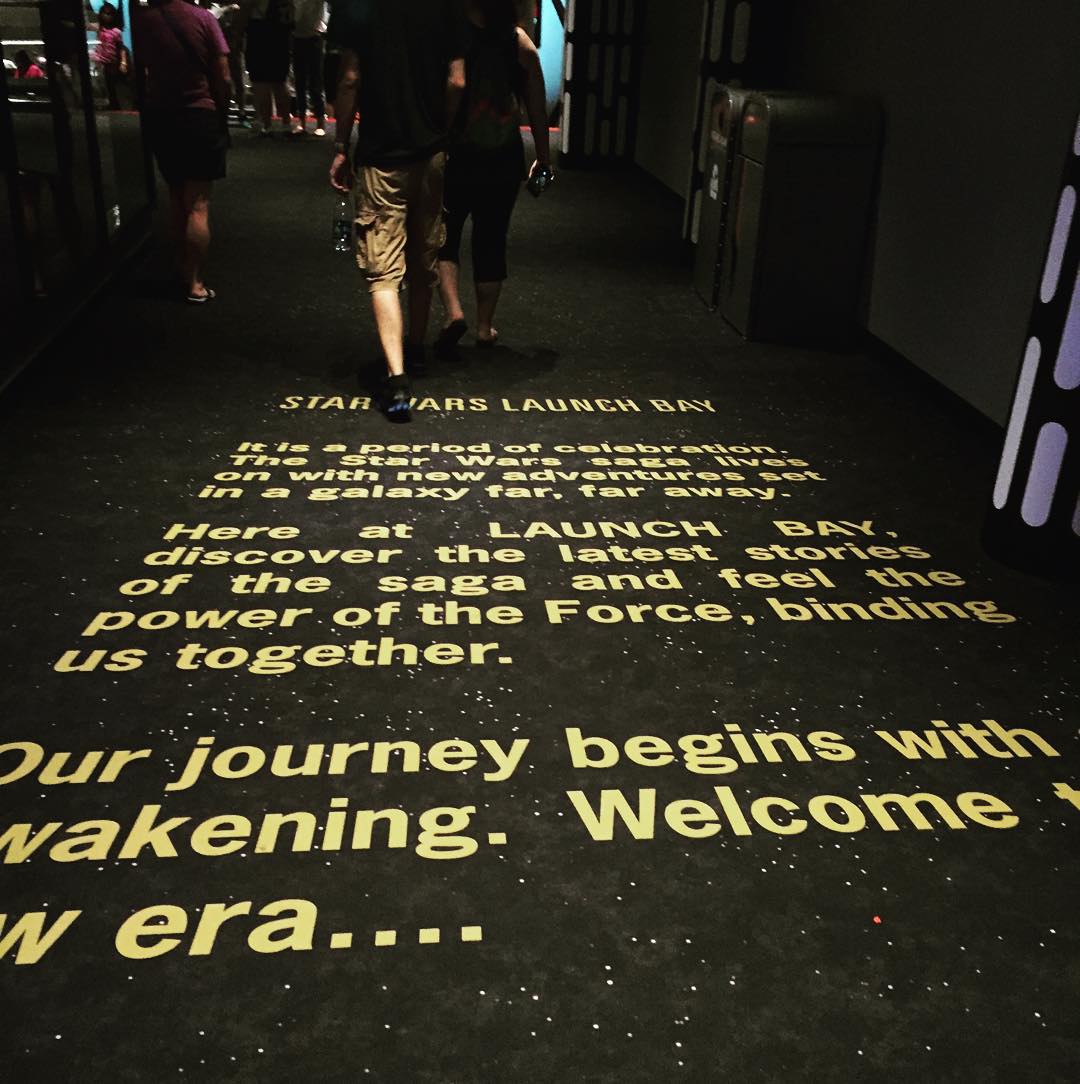This detailed, color photograph captures the lobby of what appears to be a movie theater, likely themed around Star Wars. The main focal point is the dark carpet adorned with text and stars, reminiscent of the iconic Star Wars opening crawl, complete with perspective typography that diminishes into the distance. The gold lettering on the black carpet reads, "Star Wars Launch Bay. It is a period of celebration. The Star Wars saga lives on with new adventures set in a galaxy far, far away. Here at Launch Bay, discover the latest stories of the saga and feel the power of the force binding us together. Our journey begins with awakening. Welcome to a new era." Towards the top left center of the image, several people are visible, walking away from the camera, seemingly heading towards an event or further inside the venue. The dark, indoor environment contributes an atmospheric and immersive feel, transporting onlookers directly into the Star Wars universe.